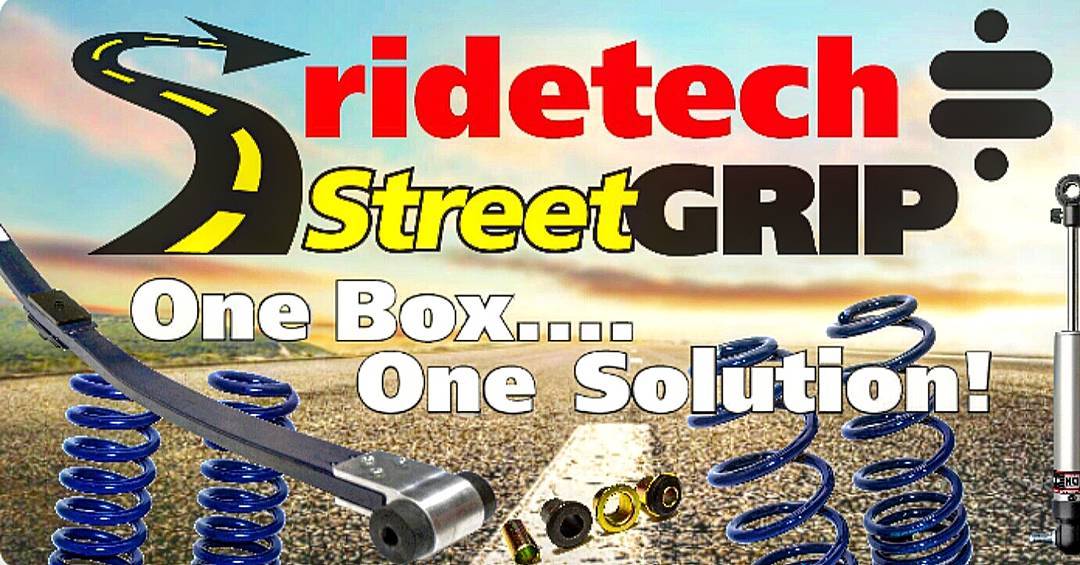The advertisement features a vibrant and detailed layout for automotive, bicycle, or motorcycle parts. In the background, there's a digitally-rendered scene of a street with visible pavement on the right and a grassy area on the left. Above the street, the sky transitions from rich blues to deep oranges and yellows, suggesting either a sunrise or a sunset. Prominently displayed in the forefront are several metallic parts, including blue coils, screws, bolts, and various fasteners, photographed sharply against the background.

The text at the top of the image is colorful and bold. In red letters, it announces "RIDE TECH," followed by "STREET" in yellow, and "GRIP" in black. White text further down the image emphasizes the product slogan: "One Box, One Solution." In the upper corners of the advertisement, minimalist logos are present; the upper right corner features a black symbol resembling an equals or division sign, while the upper left corner showcases a curved street with an arrowhead pointing forward, reinforcing the theme of movement and technology.